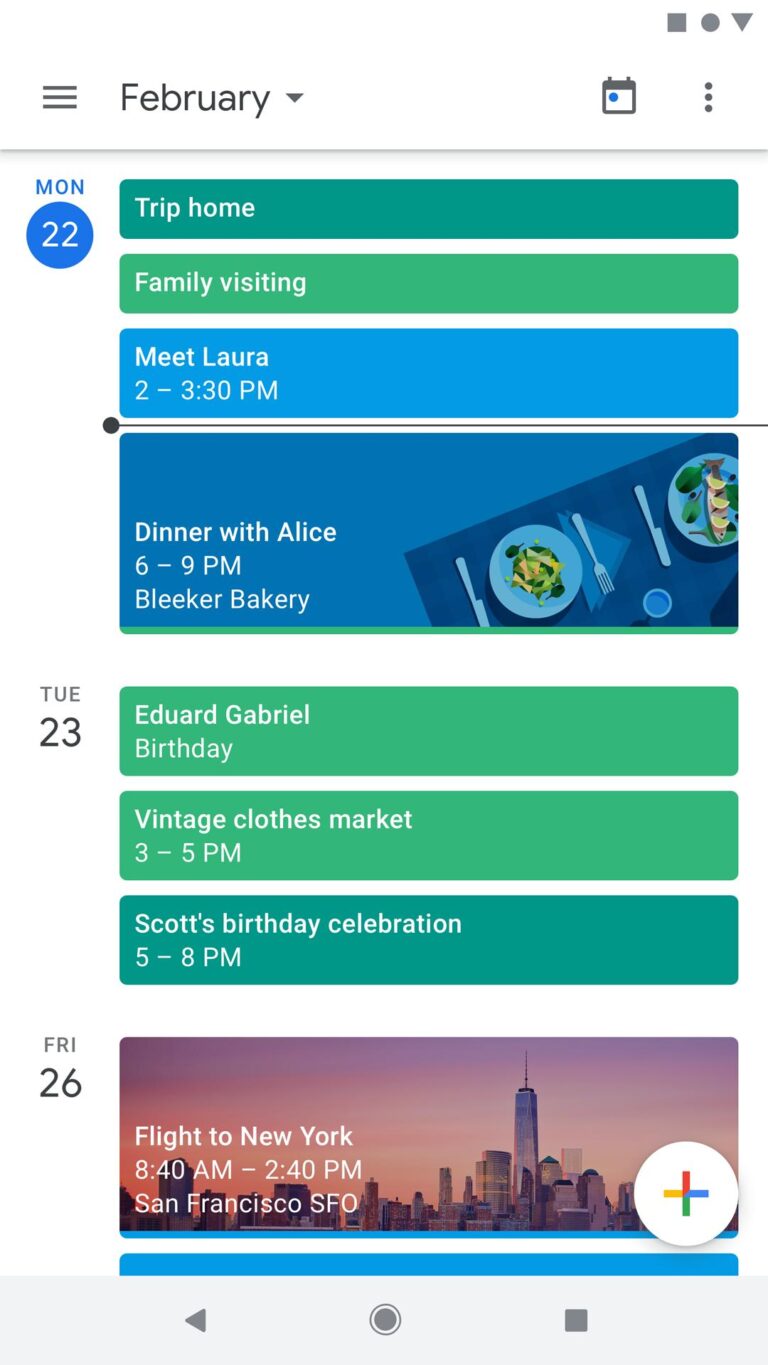The image appears to be a detailed view of a digital calendar, likely displayed within a mobile app interface. 

On the left side of the screen, there are three horizontal black bars stacked on top of each other, indicating a menu or hamburger icon, followed by the word "February" and a pull-down menu. Adjacent to this is a calendar icon and three dots stacked vertically, suggesting additional options.

Below this section, the date "Monday 22" is prominently displayed. The schedule is organized with colored bars representing different events, all with white font. A dark green bar is titled "Trip home," followed by a light green bar labeled "Family visiting." There is a blue bar for the event "Meet Laura, 2-3:30pm." Further down, a black bar is present, followed by a darker blue bar for "Dinner with Alice, 6-9pm" at Bleaker Bakery.

The next date, "Tuesday 23rd," includes a light green bar for "Edward Gabrielle, birthday" and another light green bar for "Vintage clothes market, 3-5pm." That day's schedule also includes a dark green bar for "Scott's birthday celebration, 5-8pm."

On "Friday 26th," there's an entry for a "Flight to New York, 8:40am-2:40pm" departing from San Francisco International Airport (SFO). This section is visually enriched with a photo of the San Francisco skyline in the background.

On the right side of the screen, there is a white circle with an 'X' inside, stylized with Google colors (red, yellow, blue, and green), indicative of adding a new event. Below this icon, a blue bar features navigational symbols: a backward arrow, a circle, and a square, likely representing common app controls for navigation and interface interaction.